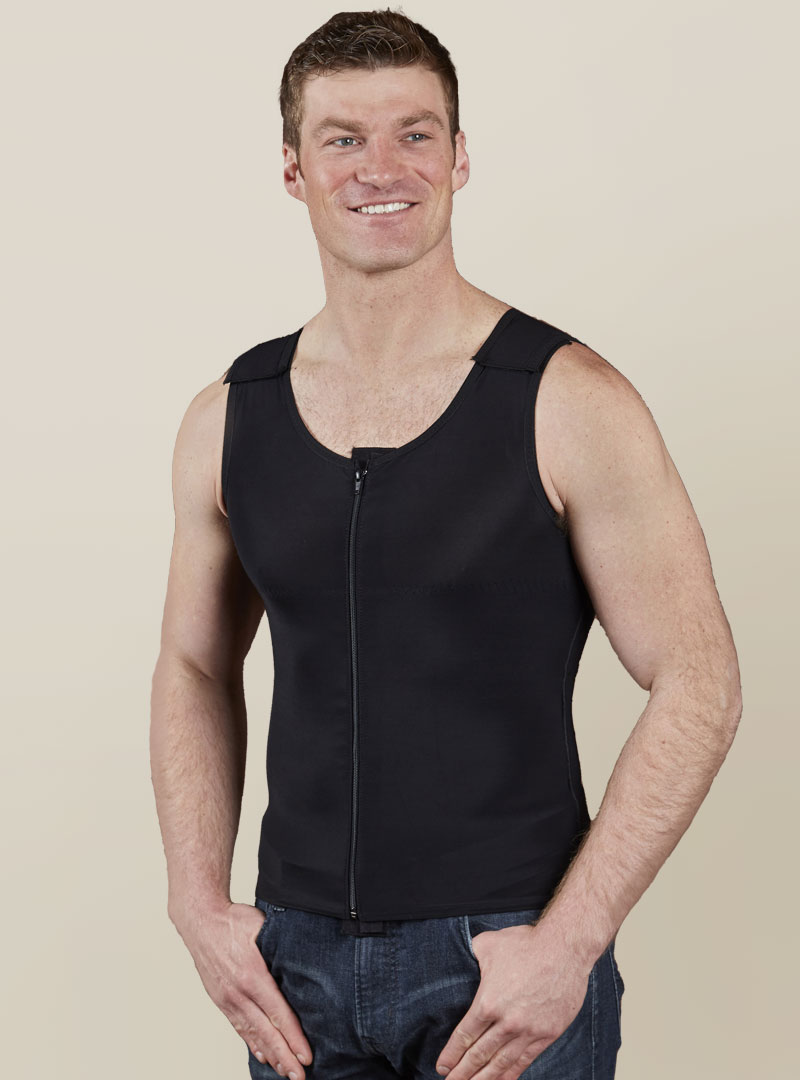In this image, we see a tall, muscular man standing against a plain tan background, with his thumbs hooked into the front pockets of his dark wash blue jeans. He is dressed in a sleeveless, black zippered vest that allows a glimpse of his toned arms, abs, and pecs, hinting at a regular workout routine. The man, who is posing as if for a professional photoshoot or magazine spread, has short brown hair and blue eyes, and he wears a slight, pleasant smile that reveals the top row of his teeth. His stance is slightly angled, with one shoulder set a bit farther back than the other, and he is looking off to the right, not directly at the camera. The background is devoid of any signs or text, ensuring the focus remains entirely on him.